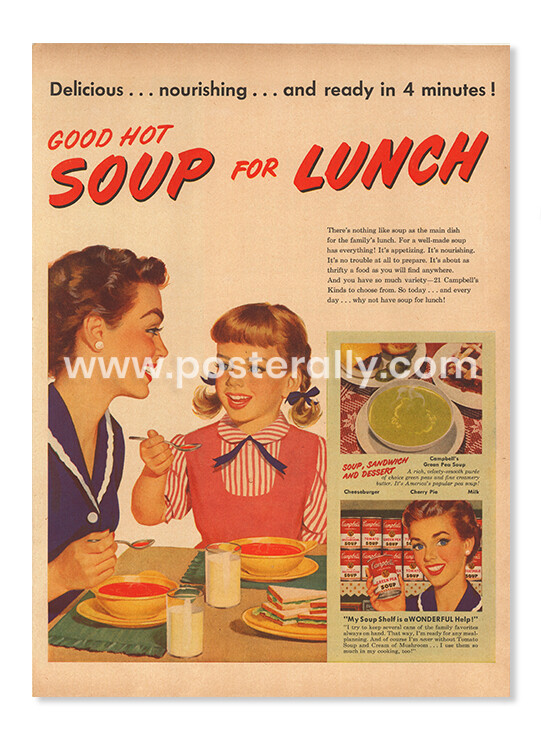The image is an old magazine cutout, likely from the 1940s or 50s, featuring an advertisement for Campbell's soup. The paper has a white, pinkish, or brownish tint. At the top in black font is the phrase "delicious... nourishing... and ready in four minutes!" Below, in bold red capital letters with a black shadow, it declares "GOOD HOT SOUP FOR LUNCH."

The right side of the image displays smaller text extolling the virtues of soup, describing it as appetizing, nourishing, easy to prepare, and economical, with a variety of 21 Campbell's kinds to choose from. The text suggests, "So today... and every day... why not have soup for lunch!"

Central to the advertisement is a large image of a woman and her daughter enjoying lunch. The mother has brown hair, blue eyes, is wearing a blue dress with white piping, and holds a can of Campbell's soup. The young girl beside her has blonde pigtails tied with blue ribbons, a red dress, a red and white striped shirt, and a blue bow at her collar. They are seated at a table with two yellow bowls filled with red soup, two glasses of white milk, and a yellow plate adorned with sandwiches that reveal hints of green filling.

To the right are two smaller images: one featuring a cup of green soup, likely pea soup, and the other showing the mother holding a can of Campbell's soup. A website, www.posterrally.com, is overlaid on the image, indicating its source.